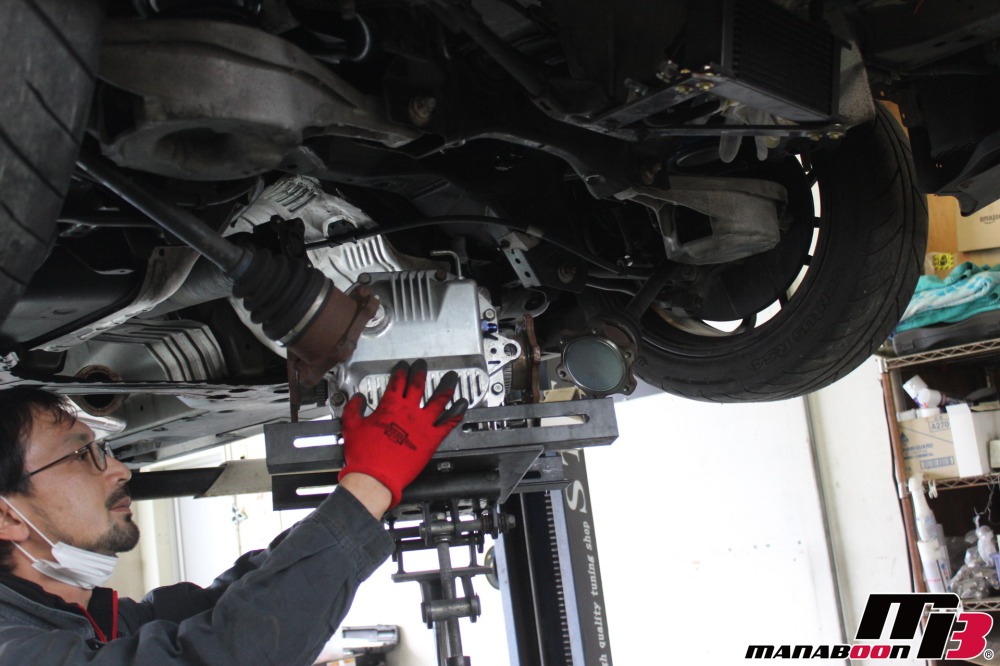Inside a bustling garage, a detailed image captures the scene from beneath a car suspended by a hydraulic lift. Dominating the foreground is an immaculately clean, chrome-finished engine being hoisted, likely to be installed into the vehicle. To the left, a focused mechanic with black hair, a mustache, and a goatee, all while wearing glasses, tends to the task. Resting around his neck, the mechanic has a surgical mask, with its ear straps loosely hanging. He is dressed in a dark gray jacket accented with a black and red collar and red work gloves, which show evident signs of heavy use with greasy stains. Nearby, the car's tire and a tangle of cables and bolts are visible, underscoring the mechanical intricacies involved. On the right side of the image, a cluttered shelf holds rags and various boxes, their contents uncertain but essential to the workspace. The garage's wall and part of the car lift frame the scene, with the bottom right corner bearing the label "Manaboon M3," indicating the car model or the lift's brand.